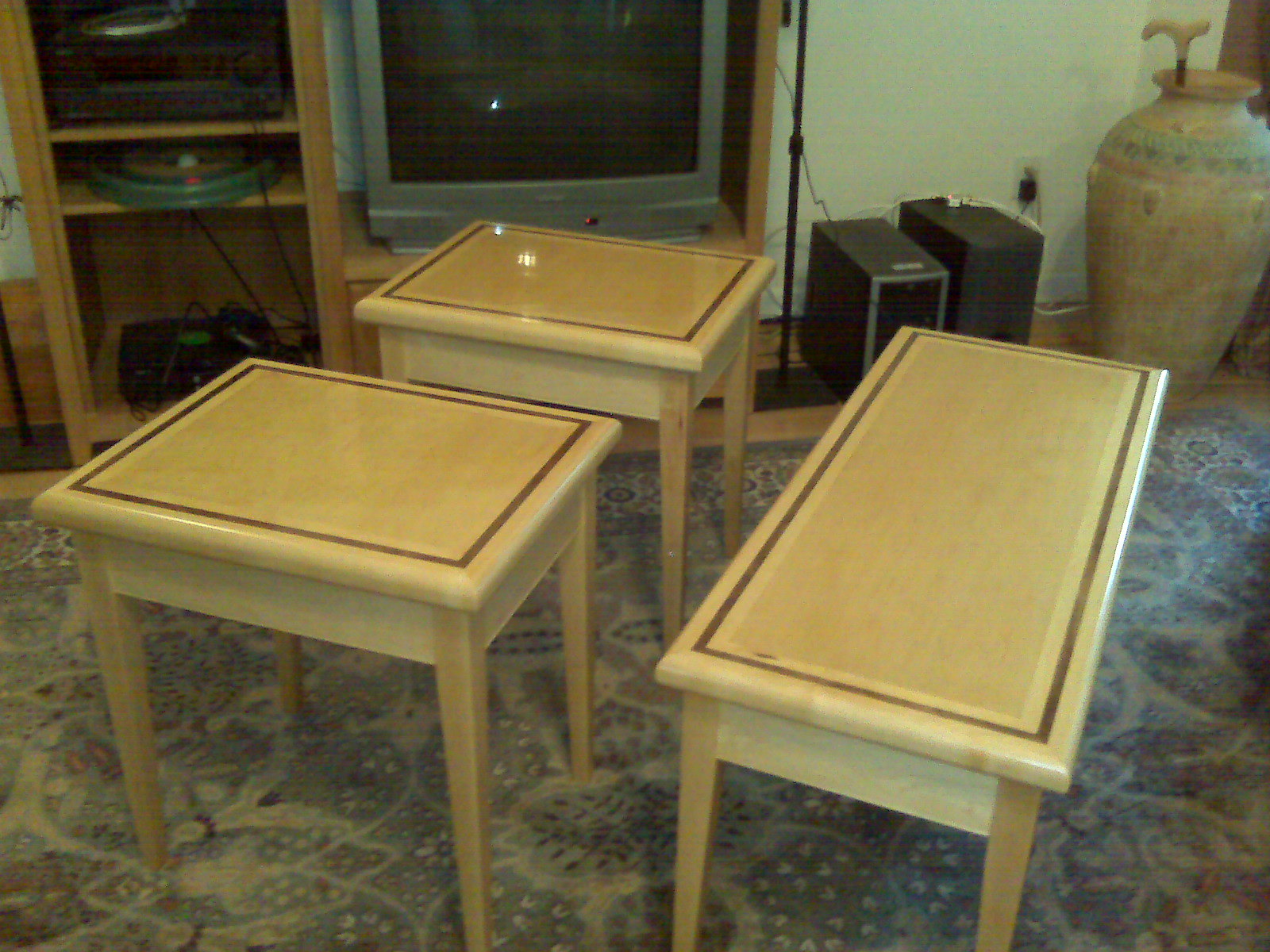The image depicts a room with three matching tables arranged on a floral-patterned carpet. The tables consist of two small, square end tables and one longer coffee table, all crafted from light wood. Each table features a distinct darker brown border accentuating the top surface. The setting appears to be someone's living room, characterized by an entertainment center in the background. This wooden entertainment unit houses a vintage silver CRT television with a dark screen. Additionally, the unit has multiple shelves holding various items, including black AV equipment, a green round object, and an original Xbox system. On the floor beside the entertainment center are two black computer towers or subwoofers. A tall, terracotta vase with whitewash and faint green, blue, and red stripes is stationed in the room's upper right corner. The vase contains a walking cane with a white hand grip. The overall ambiance is indoors and furnished in warm, tan tints, though the photograph appears slightly low in quality.